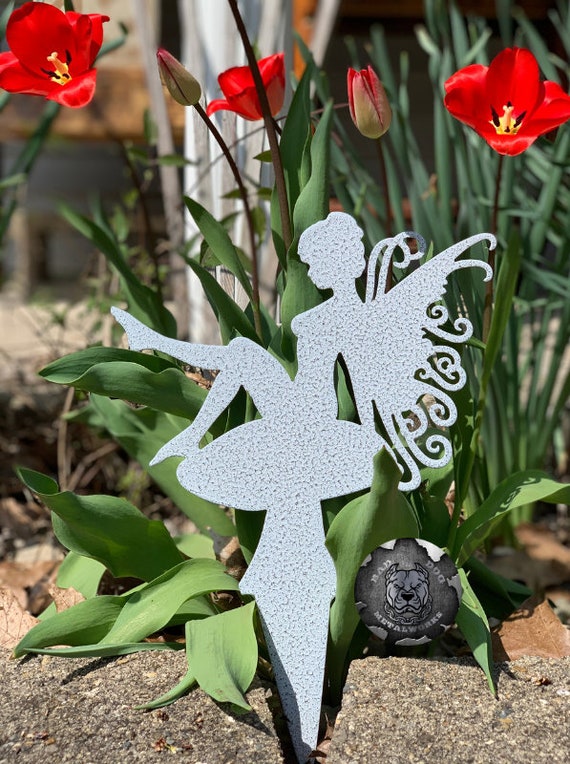The photograph captures a charming garden scene from a unique, low-angle perspective close to the ground. At the center of attention is a small metal silhouette of a fairy, reminiscent of Tinkerbell, gracefully perched on a mushroom. This delicate fairy, with her legs up and wings spread, is nestled between two stones. The metal appears to be a light gray, blending subtly with its earthy surroundings.

In the background, a vibrant plant emerges from a crack in what seems to be a cement surface, adding an element of resilience and natural beauty to the scene. This plant features strikingly bright red flowers with attractive yellow centers, contributing to a visually arresting depth of field. These blossoms appear at the top of the image, with fully open flowers on the left, middle, and right, and closed buds interspersed.

To the right of the fairy, there's a distinct painted rock depicting a bulldog, contrasting with the fairy’s ethereal appearance and adding an artistic touch. The scene is completed with a badge at the bottom right corner, labeled "Mad Dog Metalworks," hinting at the craftsmanship involved in the garden layout. Tall grass and additional green leaves frame the background, reinforcing the sense of a lush, vibrant garden taken during daylight. 

Overall, this detailed close-up offers a whimsical and vibrant portrayal of garden life, harmoniously blending natural and crafted elements.